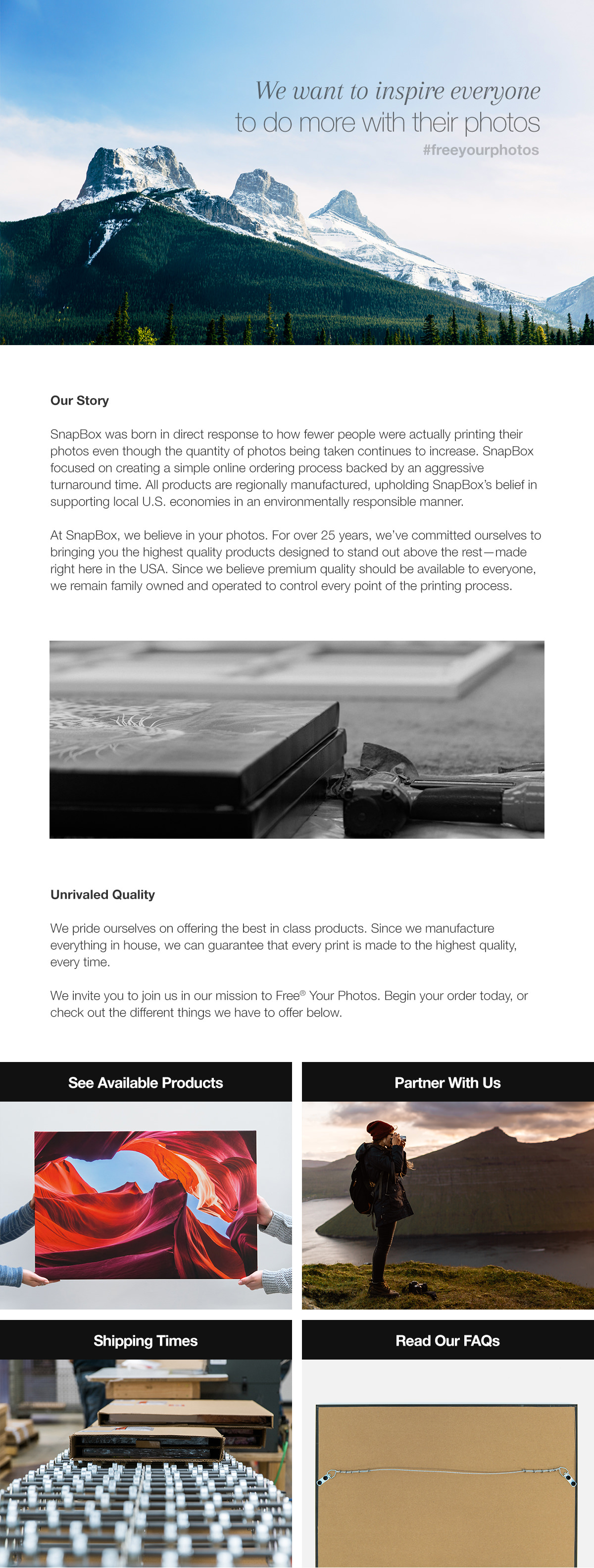This is a detailed, descriptive caption for the given image:

The screenshot displays a meticulously designed webpage. At the very top, a captivating photograph showcases a majestic snowy mountain range with three prominent peaks blanketed in snow. The base of the image is adorned with verdant conifer trees, adding a touch of lush greenery to the serene winter landscape. Above the peaks, a cloudy blue sky stretches out, providing a tranquil backdrop. Superimposed on the sky in bold black font is an inspiring message: "We want to inspire everyone to do more with their photos. #FreeYourPhotos."

Immediately below the photo, the webpage transitions to a clean white background with black font, presenting a section titled "Our Story." However, the text of the story is too small to be legible in the screenshot. Further down, there is an intriguing, somewhat eerie photo of what appears to be a broken gray tombstone, adding an element of curiosity.

Beneath this unusual image, the text reads "Unlimited Quality," followed by an illegible paragraph due to the small font size. At the bottom of the screenshot, four neatly arranged squares are visible, each topped with a black bar and labeled in white font. The options provided are "See Available Photos," "Partner with Us," "Skipping Trees," and "Read Our FAQ."